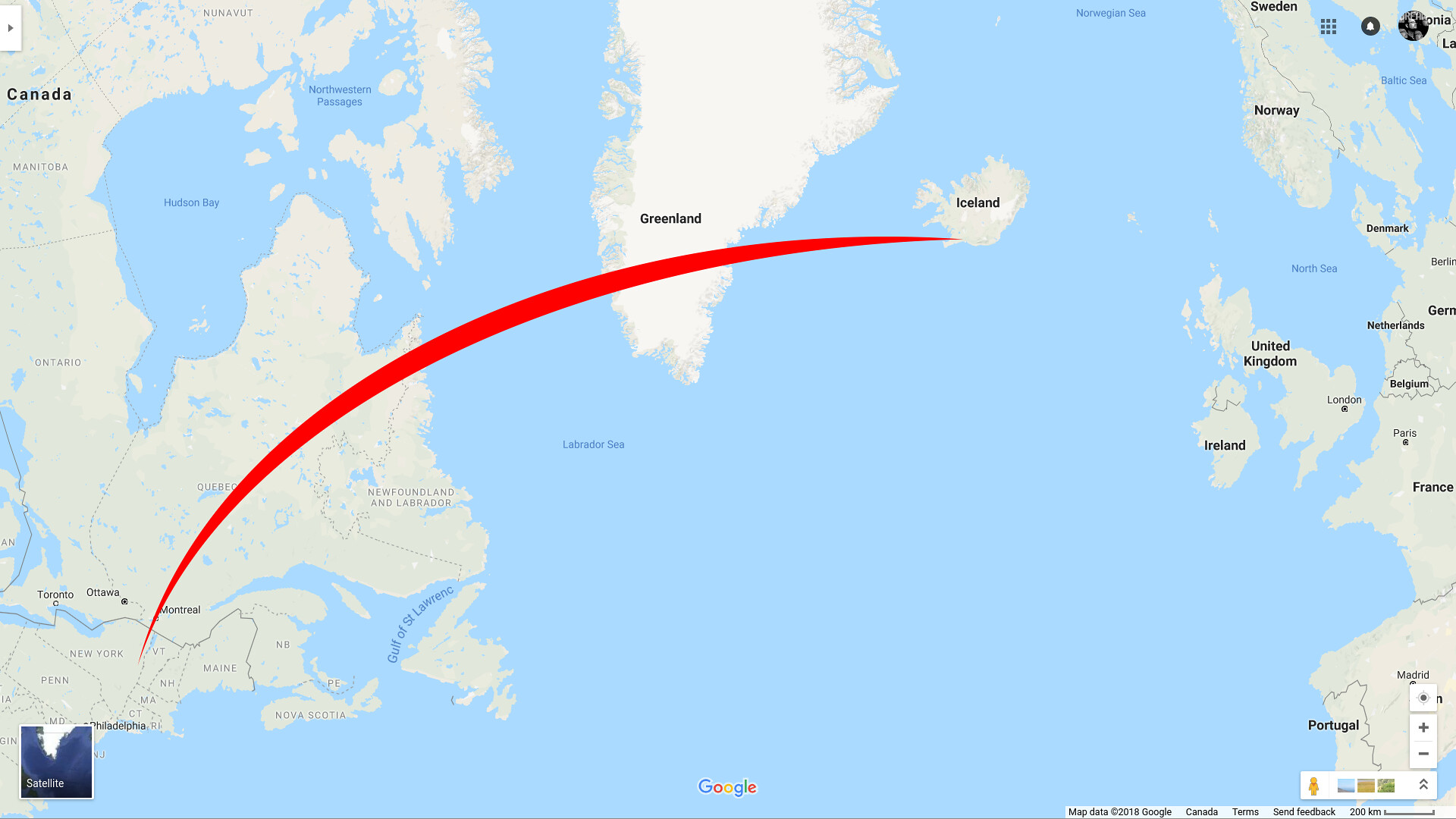The image depicts a map prominently featuring North Atlantic and surrounding regions. The map highlights Canada, Greenland, Iceland, Norway, Denmark, the Netherlands, Belgium, the United Kingdom, Ireland, France, and Portugal using black labels over a light-hued landmass. Smaller black letters indicate various cities within these countries. The eastern edge of the United States is also visible. There is a prominent red line with an arrow pointing from New York to Iceland, suggesting a route or connection between the two locations. The bottom left corner showcases a darker blue area labeled "satellite" in white letters. This section appears to represent satellite imagery or data. At the bottom right of the map, there is a gauge for adjusting the map's viewpoint, although it lacks a key to explain its specific function. Centered at the bottom is the word "Google" in multicolored letters, indicating that the map is likely sourced from Google Maps.